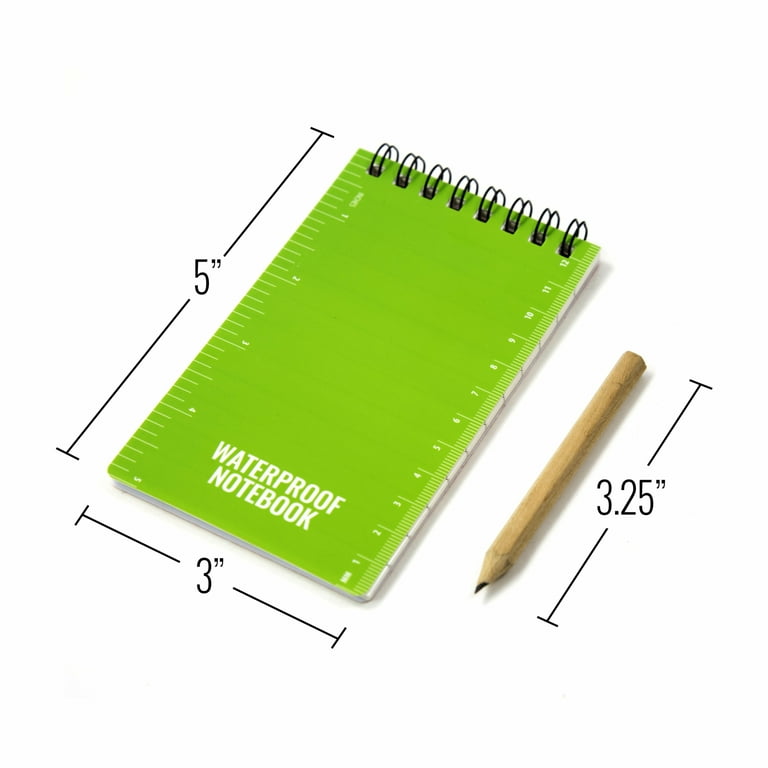The image features a detailed pixel illustration of a green, spiral-bound notebook and a wooden pencil on a featureless white surface with narrow gray shading to the right and bottom of the objects. The notebook, positioned at an angle with its bottom left corner lower and its top right corner higher, measures 5 inches in length and 3 inches in width, as indicated by black ruler-like lines on its left and bottom edges. The left side of the notebook is marked in inches, while the right side is marked in centimeters. The cover of the notebook prominently displays the text "waterproof notebook" in large white letters at the bottom. To the bottom right of the notebook lies a bare wooden pencil, sharpened and devoid of an eraser, measuring 3.25 inches in length. The precise positioning and measurements of the objects contribute to the detailed and meticulous nature of the illustration.